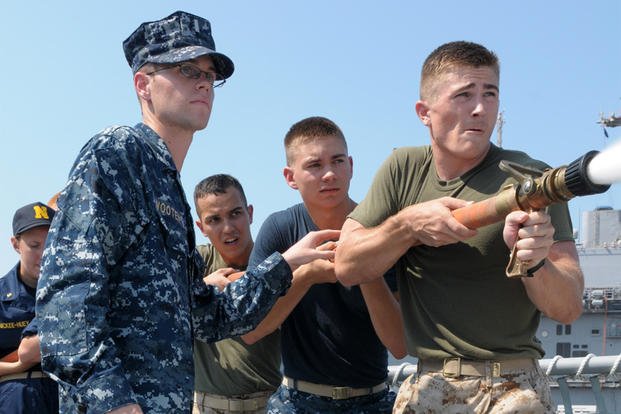In this detailed image, several individuals are engaged in a military training exercise. On the left side of the photograph, a man donning blue fatigues stands attentively. He wears glasses and a matching blue fatigued hat, indicating his readiness and focus. Centrally framed in the photo, three men firmly grip a hose as part of their coordinated effort. The man positioned at the center and the one on the far right both sport green shirts paired with brown fatigued pants, signifying uniform cohesion. The man at the center of the trio contrasts with the others by wearing a blue shirt and blue fatigued pants, adding a unique element to the group's visual dynamic. The scene vibrates with a sense of discipline and teamwork as they practice their critical skills.